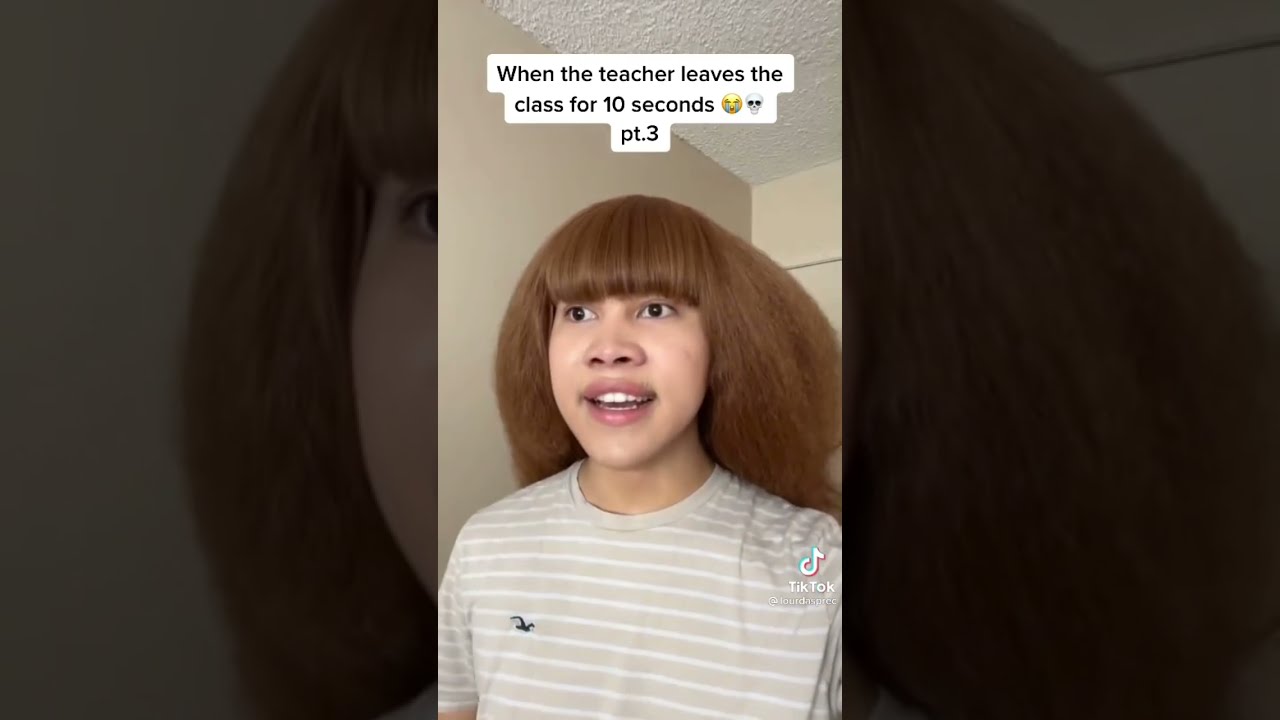This is a screenshot from a TikTok video featuring a light-skinned African American woman with red, frizzy hair and straight, curled-under bangs touching her eyebrows. She is wearing a tan T-shirt with white pinstripes and a bird logo on the right side of her chest. Her mouth is open, revealing her teeth, as if she is about to speak, and she is looking past the camera with a straightforward expression. The TikTok logo is visible on her left shoulder. The image includes a text caption at the top center in black font on a white background that reads, "When the teacher leaves the class for 10 seconds," followed by a cry emoji and a skull emoji, and below that, it says "Part 3." The portrait image is set against a darkened, enlarged background of the same image in a landscape orientation.